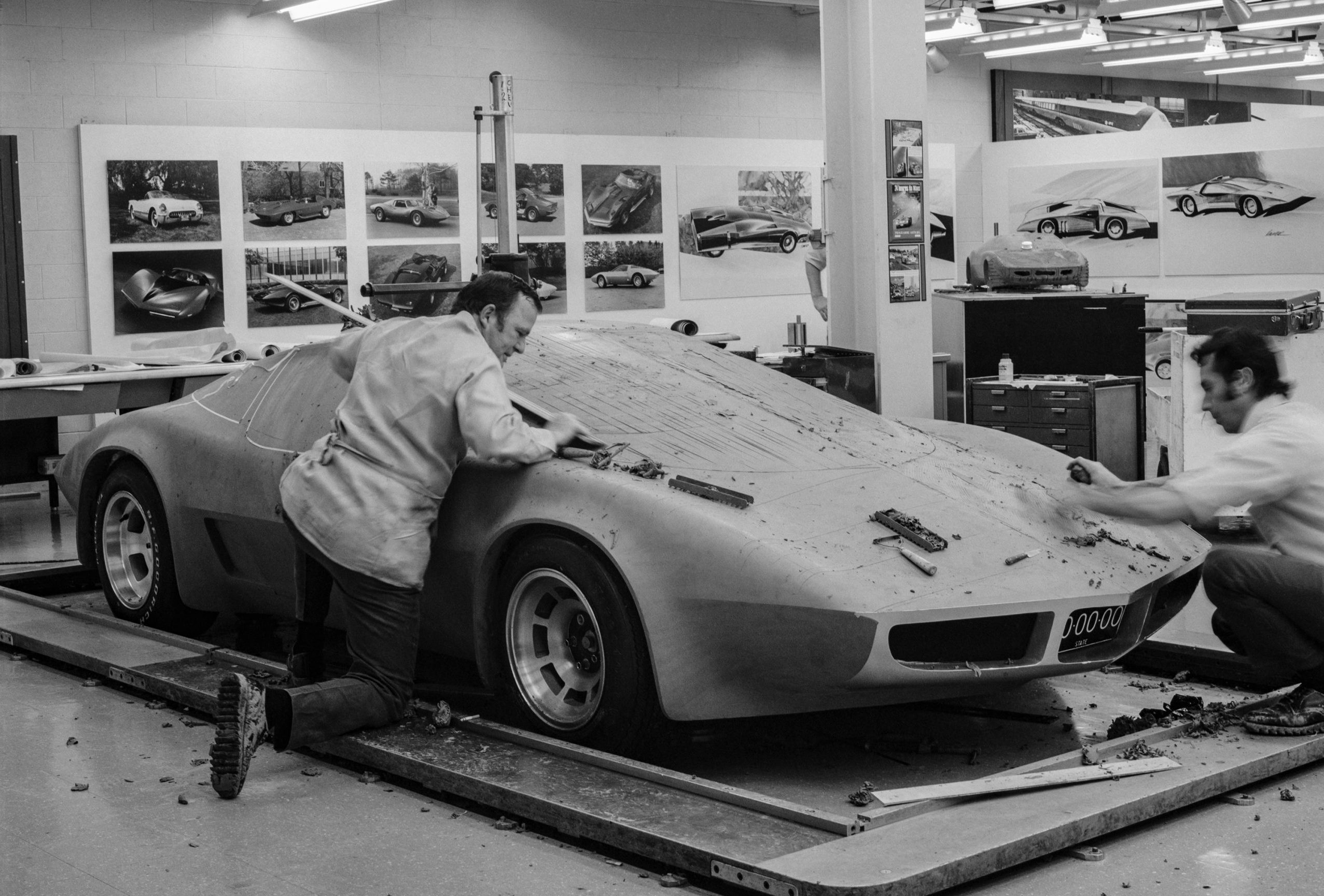In this old black-and-white photograph, likely taken in the 1960s or early 1970s, two men are diligently working on the front of an old sports car in a workshop. Both men, wearing black pants and white apron-like shirts, are engaged in what appears to be the process of shaving off parts of the car using long tools. The man on the left is kneeling, focusing intently on his task, while the man on the right's hand is a blur from his rapid movements. Shavings can be seen scattered across the car, suggesting meticulous work in progress. The indoor setting is adorned with various car-related images; photographs of cars hang on the left wall, while on the right side, there are drawings and a small model of the vehicle they are working on. A small desk is also visible to the right, adding to the detailed ambiance of a dedicated auto-repair workshop. The entire scene is rendered in shades of gray, enhancing the vintage and industrious atmosphere of the moment captured.